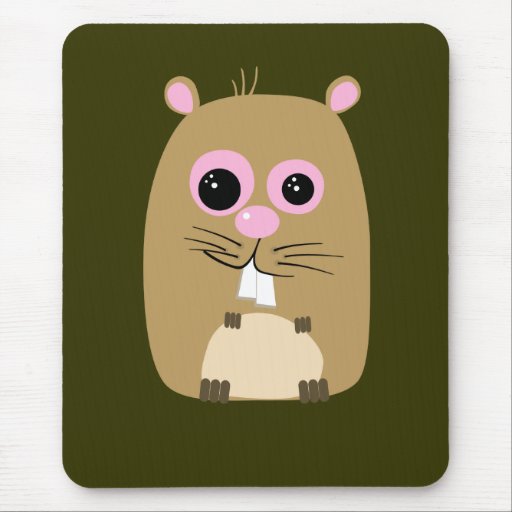This cartoon-style image appears to be a product listing for a mouse pad with a lightly textured, gray background that resembles wood. Dominating the scene is a rounded rectangular shape in dark olive green, more green than brown. At the center of this greenish-brown rectangle resides a cartoon figure of an animal, possibly a gerbil, mouse, or even a beaver. 

The character has a round, light brown face with two eyes featuring black pupils surrounded by pinkish circles. Notably, the left eye's circle is slightly larger and may appear light purple, while both eyes have a discerning pink oval nose centered beneath them. Three whiskers extend outward from each side of the nose. The creature's mouth displays two prominent white buck teeth hanging down. 

The animal's belly is a light tan color, and three short vertical lines emerge from it, suggesting feet or toes. Above the face, it has two small brown ears outlined with brown and filled with pink, accompanied by three tufts of hair sprouting from the top of its head. The overall shape of the body is an elongated oval or vertical rectangle with rounded corners, giving the impression of an adorable, cartoon animal sitting up and facing forward.